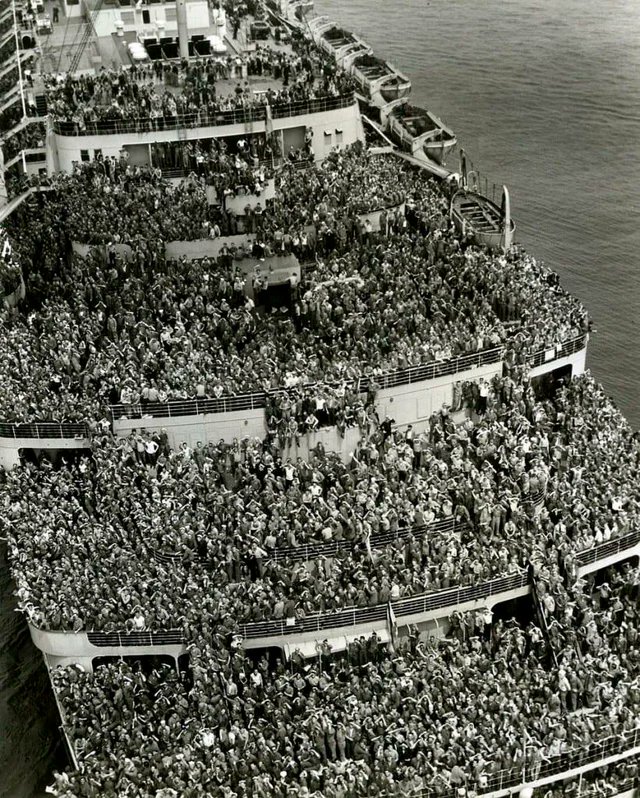This black-and-white photograph captures a striking image of a vast ship, possibly a Navy ship or a large troop carrier, densely packed with people across at least three visible decks. The ship, seemingly navigating calm waters, shows hundreds, if not thousands, of individuals clad primarily in drab clothing, with occasional white t-shirts standing out. The decks are so overcrowded that people occupy every available space, including the stairways and edges, where some can be seen sitting with legs dangling. Lifeboats hang off the sides and back of the ship, underlining the sheer scale and potential emergency preparedness of the vessel. Despite a few scattered lounge chairs suggesting a semblance of leisure, the overwhelming presence of densely packed individuals bespeaks a more critical purpose, be it a military operation or a large-scale evacuation.